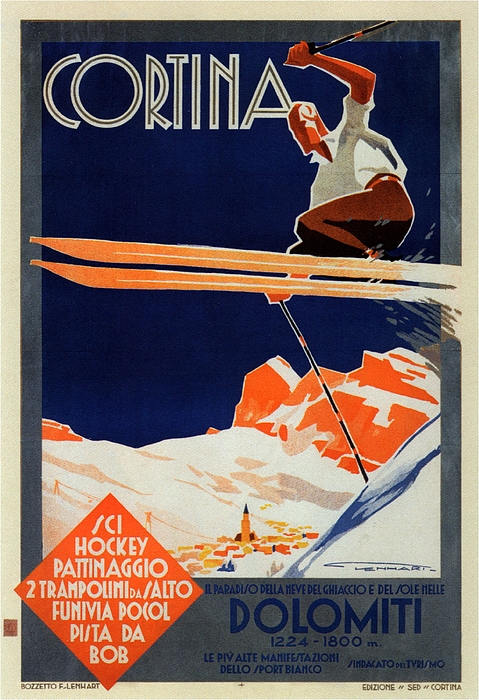This image depicts a vintage-style advertisement poster for a ski resort, likely located in Italy. Dominating the upper section of the poster, the word "Cortina" is prominently displayed in large, gray and white letters. The central illustration is a dynamic, graphic art representation of a skier soaring through the air. The skier is dressed in brown pants and a white shirt, with striking orange skis. The background features a blue sky and stylized orange mountains, creating a vivid and vibrant scene with a 3D cartoon-like quality. In the lower right section of the poster, an orange diamond-shaped text box contains information in Italian, mentioning terms like "Hockey," "Pista de Bob," "Salta Funivia," and "Patanagio." The poster has a grayish beige border, framing the central illustration and text, emphasizing the overall vintage aesthetic.